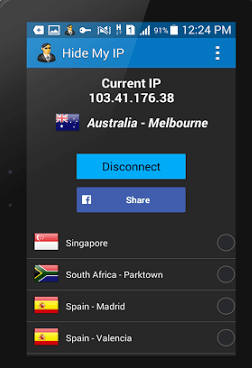The image presents a user interface with distinct elements arranged across a predominantly black background. In the top-left corner, there is a section containing various icons, including an individual wearing sunglasses and a suit, suggestive of a professional or security-themed image. The person has short hair and a blue tie, enhancing the formal depiction.

Adjacent to this, a pictogram of a key is visible, coupled with a non-audio speaker symbol, labeled with the letter "H". Below these icons, digital signals and numerical indicators, such as "91%" and "12:24 p.m.", are displayed, possibly representing network or connectivity status.

Further details reveal text fragments "hi my IP" along with an IP address formatted as "103.4.0.76" and "138". The interface includes national flags representing different countries: a prominent feature of a British or Australian flag, a blue rectangular button labeled "Disconnect", and a dark blue "Share" button for social media or Facebook interaction. Additionally, the iconography includes a Singaporean flag (red on top, white on the bottom), followed by informational nodes denoted as "Notre".

Various flags from South Africa (Parktown), Spain (Madrid and Valencia), with the colors red, yellow, and red, punctuate the display, alongside channels or columns described as "line, line, line, line."

Overall, the caption elucidates a sophisticated and multi-faceted digital interface with a plethora of geographical indicators and connectivity tools, hinting at an application designed for managing network connections or virtual private networks (VPNs).